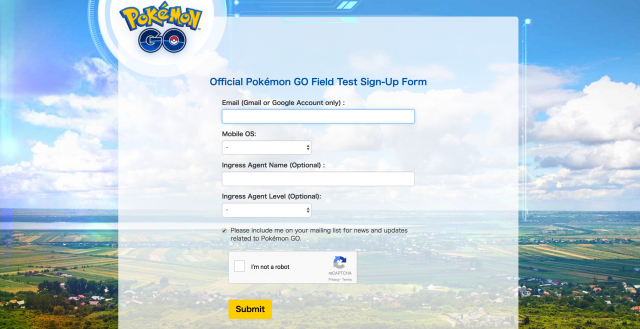The image depicts a sign-up form for the official Pokémon GO field test, set against a picturesque background. 

Against the backdrop of a sprawling, scenic landscape featuring endless acreage, a serene waterway in the distance, and a canvas of beautiful blue skies adorned with picturesque clouds, the Pokémon GO logo is prominently positioned on the left side.

Overlaying this idyllic scene is a pop-up box labeled "Official Pokémon GO Field Test Sign-Up Form." The form comprises four vertically arranged input fields:

1. **Email** (Gmail or Google account only)
2. **Mobile OS** with a dropdown menu for selecting the operating system
3. **Ingress Agent Name** (optional)
4. **Ingress Agent Level** (optional) with a corresponding dropdown menu

Additionally, there is a checkbox labeled "Please include your making first for needs of updates," possibly requiring clarification. 

The form also includes a CAPTCHA to confirm "I'm not a robot," followed by a prominent yellow "Submit" button at the bottom.